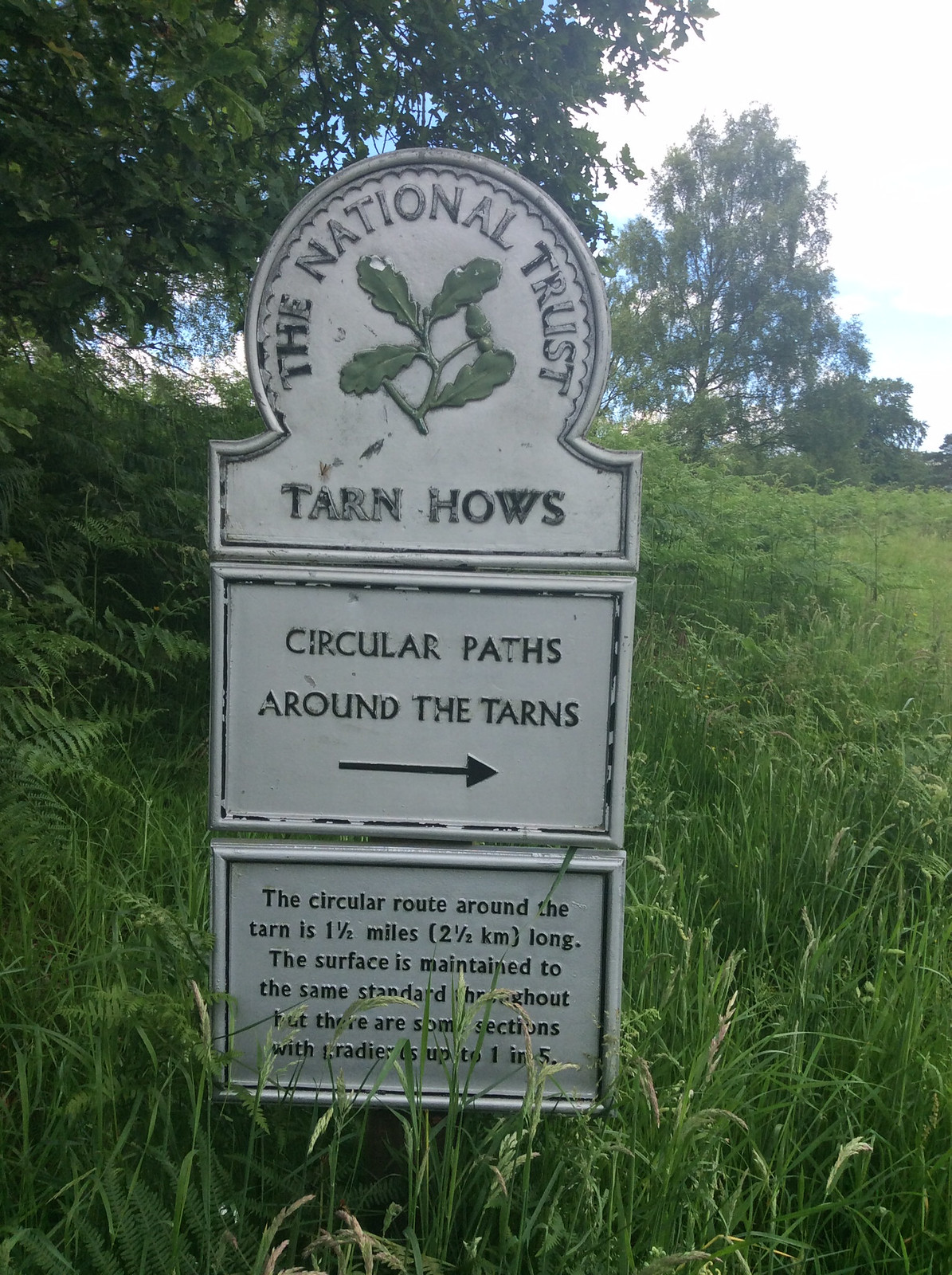The image features an outdoor sign situated in the middle of overgrown grass with trees visible in the background under a partly cloudy sky. The sign is gray with green writing and contains the National Trust logo, which includes a depiction of green leaves. The top of the sign reads "The National Trust Tarn House." Below this, it states, "Circular path around the tarns," accompanied by an arrow pointing to the right. The sign also contains a paragraph describing the route: "The circular route around the tarn is 1.5 miles (2.5 kilometers) long. The surface is maintained to the same standard." Some words are obscured by the surrounding grass. The predominant colors in the image are green and white, with a mix of blue and white in the sky.